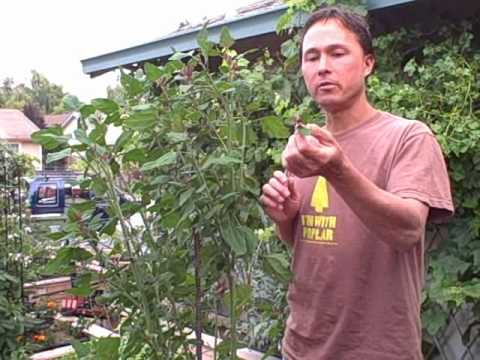The photograph shows a man standing outdoors in an urban garden setting near his house. The image, slightly blurry and compressed as if it were a thumbnail from a YouTube video or a video screenshot, captures the man on the center right wearing a light pink t-shirt with the yellow text "I'm with poplar" and an arrow pointing upwards toward a tree graphic. The man has short brown hair and is holding a large green leaf in his left hand, possibly inspecting it. To his left, several tall plants with long thin stalks and lush green leaves are growing, either from the ground or in wooden boxes that seem to be part of a garden area. Behind him, a roof awning with a gutter extends out from the upper right corner of the image, indicating the edge of a building. Further in the background to the left, one can see additional residential houses and a blue vehicle parked in front of them. The scene suggests that the man is tending to his garden in a space abundant with plant life amidst a neighborhood setting.